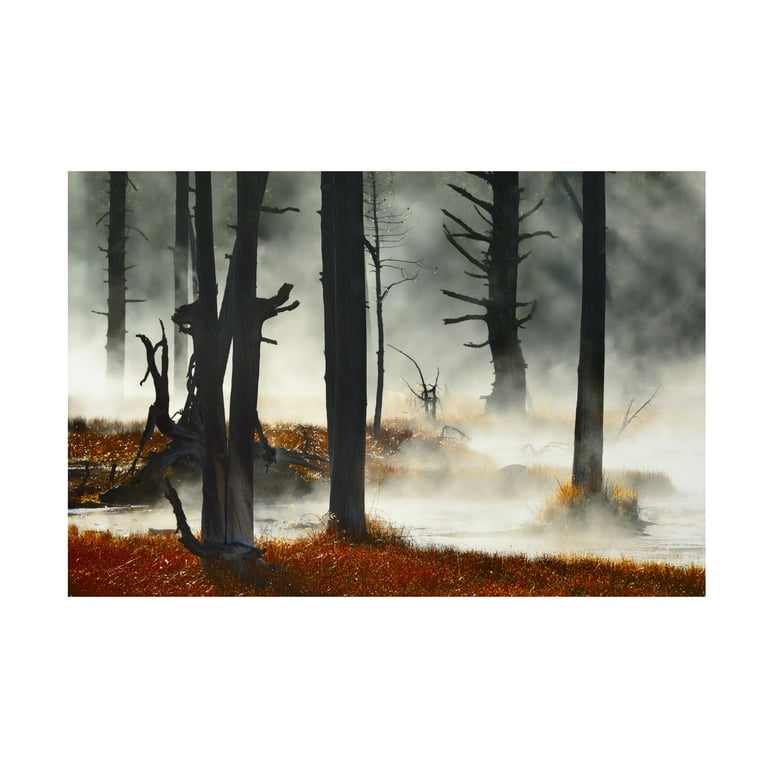An intricate and dramatic CGI or digitally-produced image captures a post-forest fire scene in a wooded area. Dominating the image are several bare tree trunks, ranging from slender to thick, with a few fractured branches extending outward. These trees rise up and disappear off the top of the frame, contributing to an eerie atmosphere. In the distance, additional trees stand shrouded in dense, wispy white smoke, which embeds a sense of mystery and desolation. The ground throughout the image is a striking reddish-orange color, possibly representing scorched earth or autumn leaves, and contrasts vividly with the stark, blackened tree trunks. The lower right segment of the scene features a foamy, silvery-blue patch of water, from which more smoke billows upwards, blending with the surrounding haze. The black clouds and the pervasive, thick white fog in the background deepen the scene's somber mood, evoking the aftermath of a fierce wildfire.